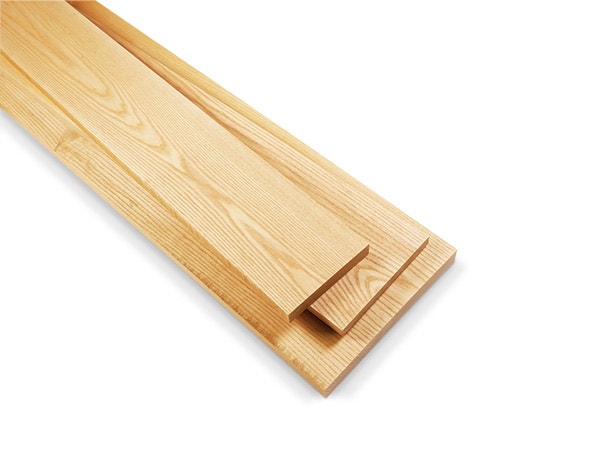This photograph features three wooden boards of light brown color with visible grain patterns, stacked on each other at a diagonal angle from the bottom left of the image. The boards differ in width, with the widest board at the bottom, a somewhat narrower board in the middle, and the narrowest board on top, slightly misaligned, creating a crooked appearance. The photo has a clean, white background and no text, giving a clear view of the boards, which look like they might be used for flooring. The precision cut of the boards suggests they were processed with a high-quality woodcutter, and though all three boards appear to be of the same length, their varying widths are the prominent feature highlighted here.